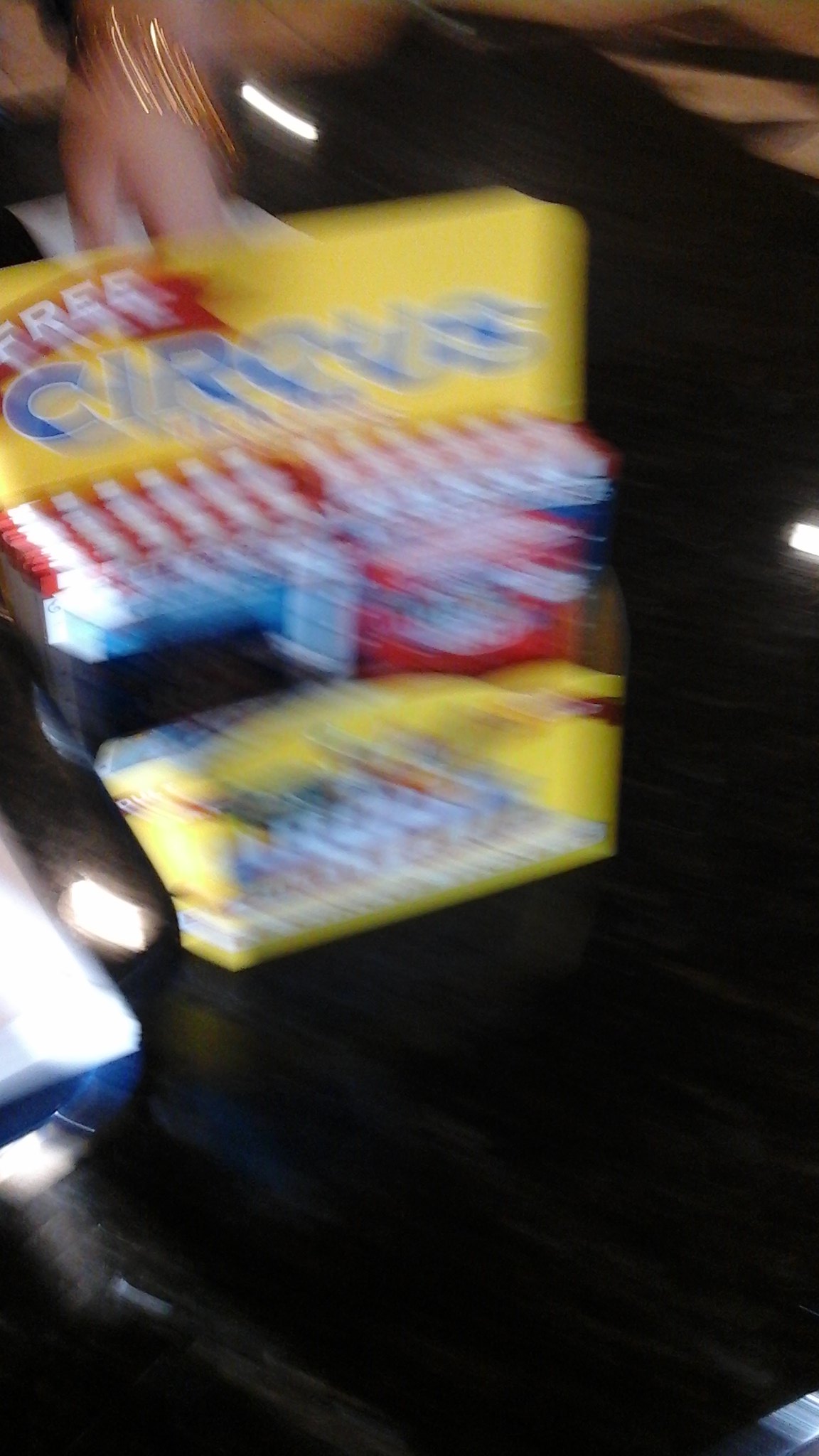A blurry photograph shows a yellow packaging at the center, possibly on a black surface like a table or a checkout counter belt. The packaging features a prominent red banner in the top left corner with the word "Free" in white text. Below the banner, in large blue text, it reads "CIRQUS." The lower section of the packaging appears to contain items with red and white striped patterns, possibly napkins or straws, stacked or standing up. There is a hand with a fair complexion and a gold bracelet visible at the top left, either holding or positioned behind the package. The surrounding area is predominantly black and largely indistinct, with reflections on the surface and a small silver corner peeking from the bottom left. There are hints of light blue and other various colors, but the overall image is difficult to discern due to the blurriness, likely caused by camera motion.